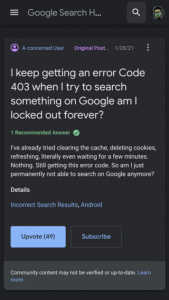A vertically oriented, narrow, low-resolution screenshot of a Google search page is displayed with a predominantly black background. The text "Google" appears in gray at the top. Below, a user named "Concerned user" has posted an issue with Google Search, specifically citing an error code 403. The user explains attempts to resolve the issue, including clearing the cache, deleting cookies, refreshing the page, and waiting a few minutes, to no avail. The post, "Original post 12121," has 49 upvotes, indicated by a blue button. There's a black "Subscribe" button below the post. The interface text appears in various colors such as gray, white, purple, blue, and green. Some text is too blurry to decipher, but it ends with the partially readable word "learn." The discussion falls under a category likely related to incorrect search results on Android devices.